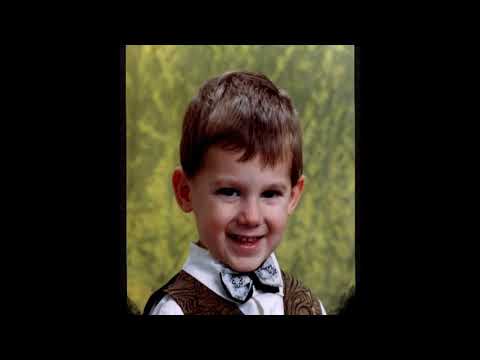This color photograph features a young white boy, approximately five years old, who exudes happiness as he smiles broadly, revealing a gap between his baby teeth. His dark eyes and short, straight brown hair frame his face, with his hair neatly pushed forward on his forehead. His ears are slightly wide, characteristic of a young child. He is dressed in a smart outfit consisting of a white button-up collared shirt, a brown vest with gold and black patterns, and a light blue bow tie adorned with designs.

The background of the image appears to be green vegetation, suggestive of an artificial backdrop typically used in professional posed photographs. The boy is positioned slightly turned to his left (our right) while facing the camera directly, reinforcing the idea of a formal setting, possibly reminiscent of a school photo.

Surrounding the central photograph is a thick black border on both the right and left sides, with a thinner black edge on the top and bottom, creating a small, square frame for the actual image. There are hints of other children's hair peeking from the bottom corners, suggesting that the original photo may have been of a larger group, and this picture was focused and edited to center on the boy exclusively.